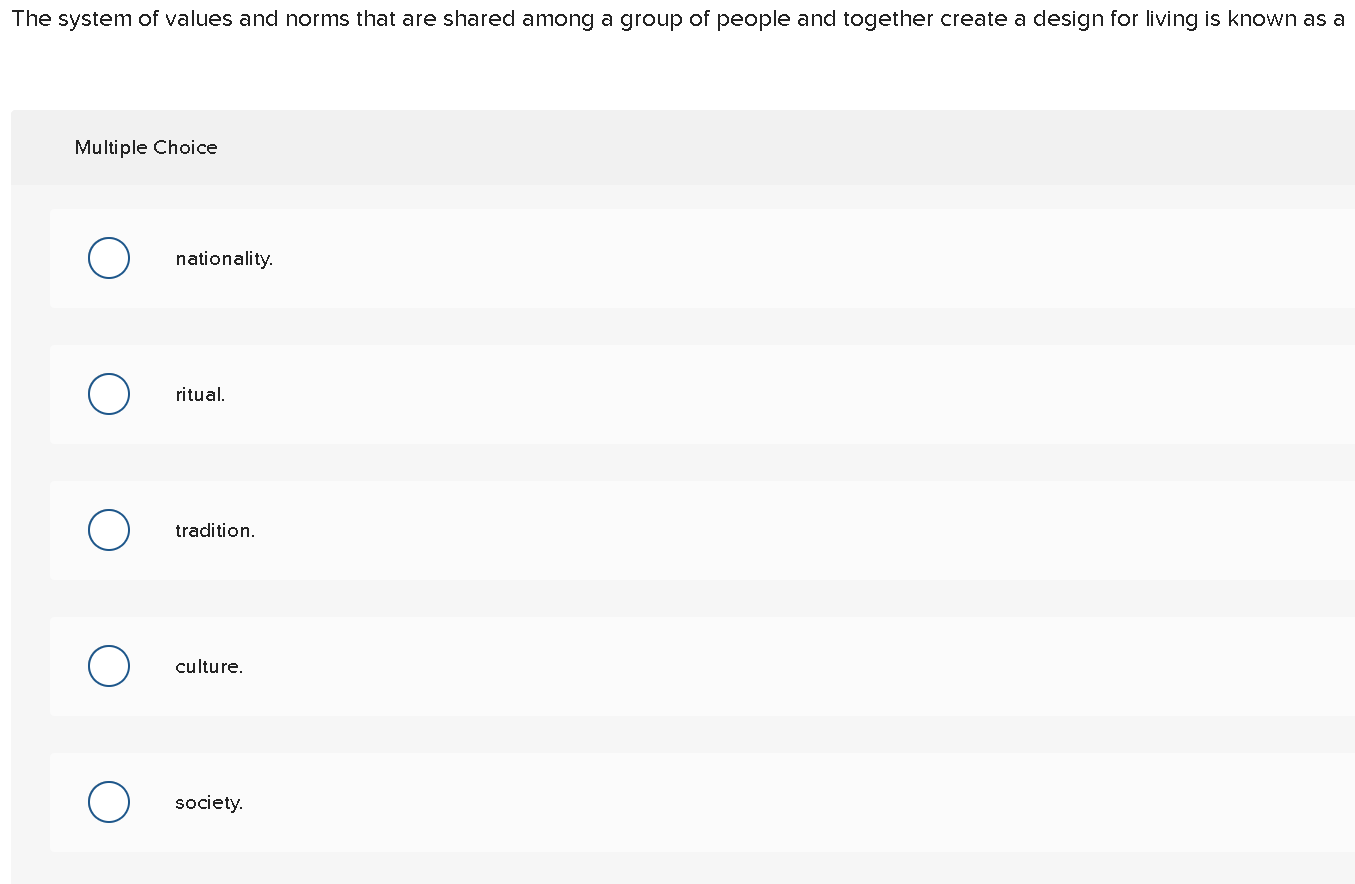The image captures a screenshot of a multiple-choice question displayed on a laptop screen. At the top, in bold black text, the question reads: "The system of values and norms that are shared among a group of people and together create a design for living is known as A." Below this, a series of five answer choices are listed vertically, each accompanied by a white dot to the left, which can be selected by clicking a blue circle. The choices provided are: nationality, ritual, tradition, culture, and society. Above the answer choices, it indicates that this is a multiple-choice question. Based on the phrasing and format, this appears to be a question from a test or quiz, likely for an academic class. The correct answer is implied to be "culture," but the person taking the quiz has not yet selected an answer.